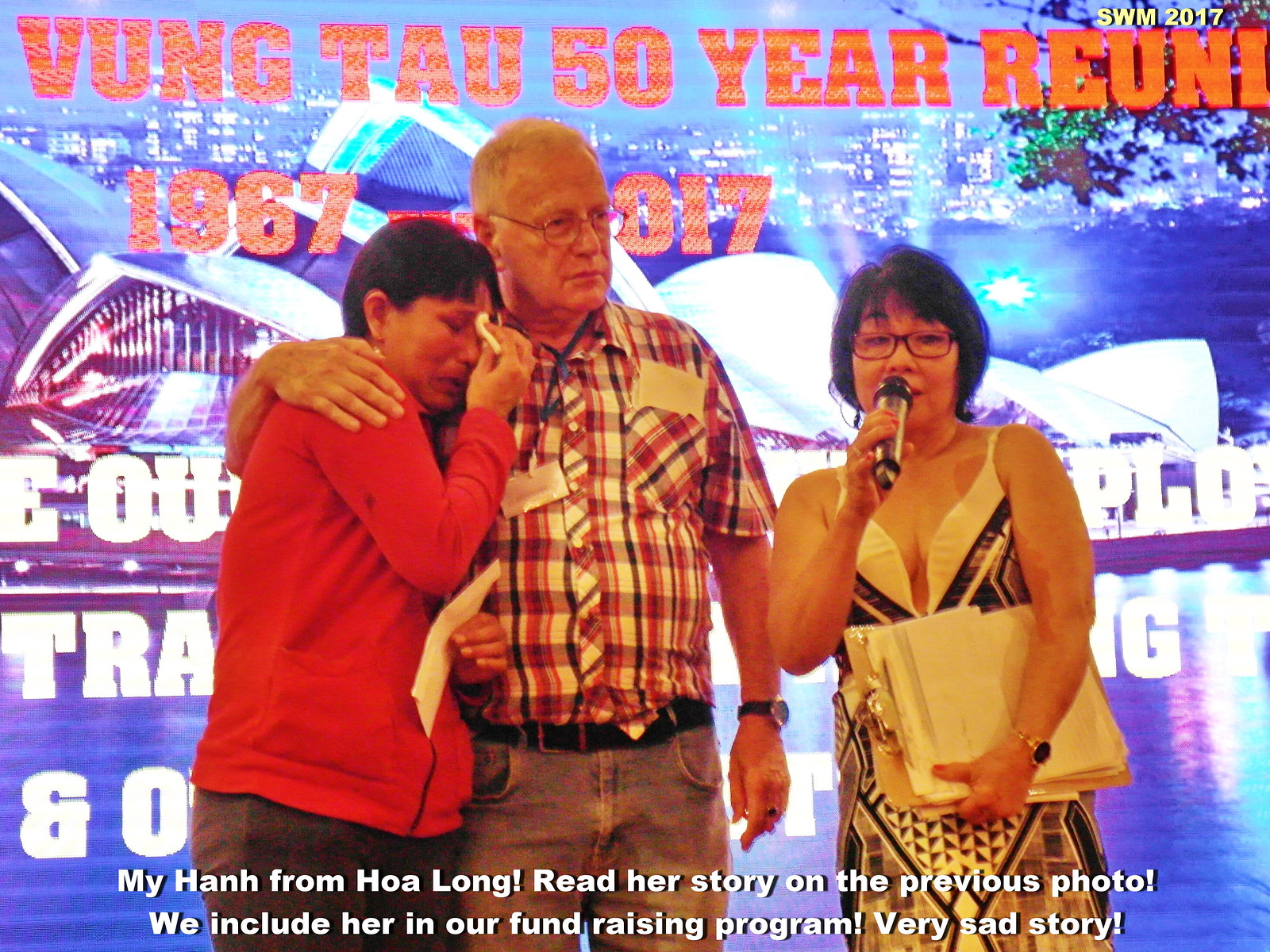In this poignant image, three individuals are prominently featured at what appears to be an indoor reunion event, specifically the "Vung Tau 50 Year Reunion 1967 to 2017," noted in red text across the top. At the center, an elderly man with gray hair, glasses, and a red plaid shirt has his arm around a woman who appears to be crying. She has short brown hair and is wearing a red sweater. To their right, a shorter woman with short black hair, dressed in a black and white outfit, holds a microphone in one hand and a white clipboard in the other, indicating she might be speaking to the audience. The background is vibrant and features an image resembling the Sydney Opera House, adding a bright blue and shiny ambiance to the scene. The lower caption on the image reads: "My Han from Ho Long, read her story on the previous photo. We include her in our fundraising program. Very sad story." The color palette in the photo includes shades of white, red, tan, maroon, brown, purple, blue, orange, green, and yellow, giving the scene a rich and varied appearance.